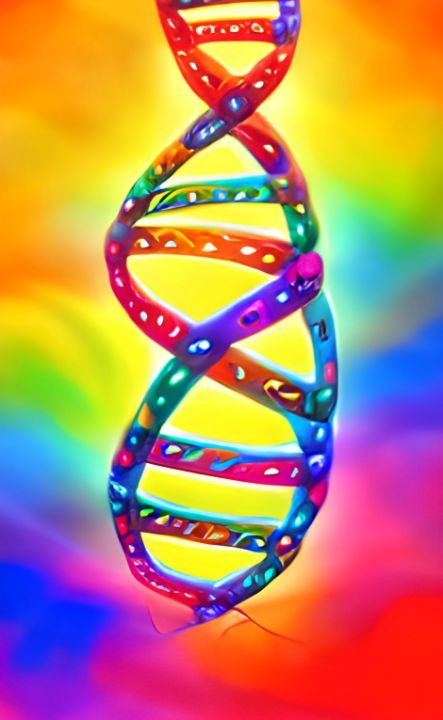The image depicts a vividly colorful and surreal scene featuring a DNA strand set against a rainbow-like background. The backdrop showcases a soft blend of colors including red, orange, yellow, green, blue, purple, and magenta, creating a smooth and harmonious gradient. In the center of the image, there is a prominent depiction of a DNA chain visualized with multiple sections that exhibit a spectrum of bright colors such as teal, pink, red, purple, and orange, arranged in a twisting, string-like manner reminiscent of medical documentaries. The DNA strand itself appears in varied shapes and sizes, enhancing the vibrant and dynamic nature of the image. Additionally, a black line is present on the bottom right, extending downwards, providing a stark contrast to the otherwise colorful composition. The overall scene is extremely colorful, bright, and visually stunning.